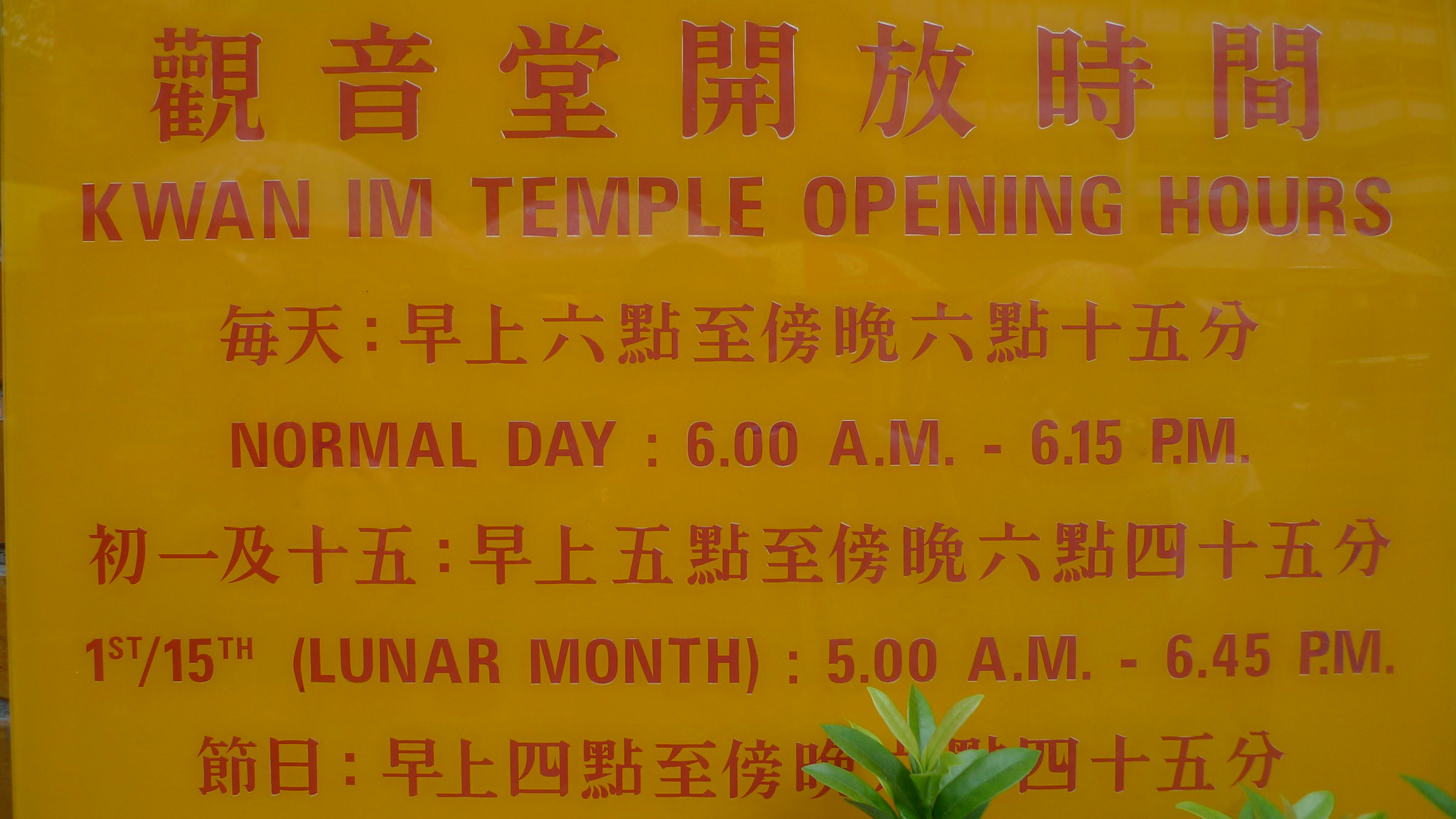The image depicts a yellow sign adorned with characters in an oriental language, prominently highlighted in red letters at the top that read "K1 IEM Temple Opening Hours." Below this title, the sign details the temple's operating hours in English: "Normal Day: 6:00 a.m. - 6:15 p.m." and "1st/15th Lunar Month: 5:00 a.m. - 6:45 p.m." Interspersed between these English lines are rows of text in a foreign language. The bottom right corner of the sign features green plant leaves, some darker and some lighter, with three sections of leaves visibly extending upwards, the center section being the tallest. The overall color scheme of the sign is goldish yellow with red lettering, creating a striking visual contrast.